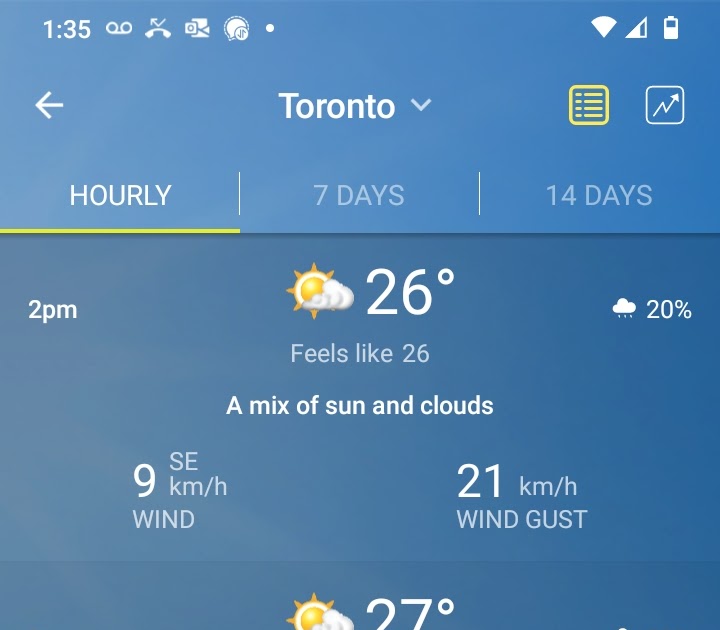The image appears to be a screenshot from a weather application on a mobile device. The interface features a blue background with white text and various informational icons. 

In the upper left-hand corner, the status bar displays the time as 1:35 along with a record icon, a divert call icon, an unidentified icon resembling a document with a square to its left, and a speech bubble icon with a small dot nearby. To the right of these icons are the Wi-Fi signal strength, mobile network strength, and a battery icon indicating it's half full.

Below the status bar, there is a navigation section with a back button on the left. The center shows the location "Toronto" accompanied by a downward arrow, likely indicating a dropdown menu for location selection. To the right, there are two icons: one square-shaped with horizontal lines in yellow, and another one resembling a graph with an upward arrow.

The main display area showcases the weather forecast. The view shows hourly weather data selected in yellow, while options for '7 days' and '14 days' are greyed out. Centrally placed is an illustration of a sun partially obscured by a cloud, indicating mixed weather conditions. To the left, it shows the time as 2 PM and the temperature as 26 degrees Celsius, with text indicating it "feels like 26." To the right, there is a cloud icon denoting a 20% chance of rain.

Further information includes wind speeds of 9 km/h from the southeast, with gusts up to 21 km/h. At the very bottom center of the image, there is a temperature reading of 27 degrees Celsius next to another partially obscured sun icon, though the lower part of this section is cut off in the image.